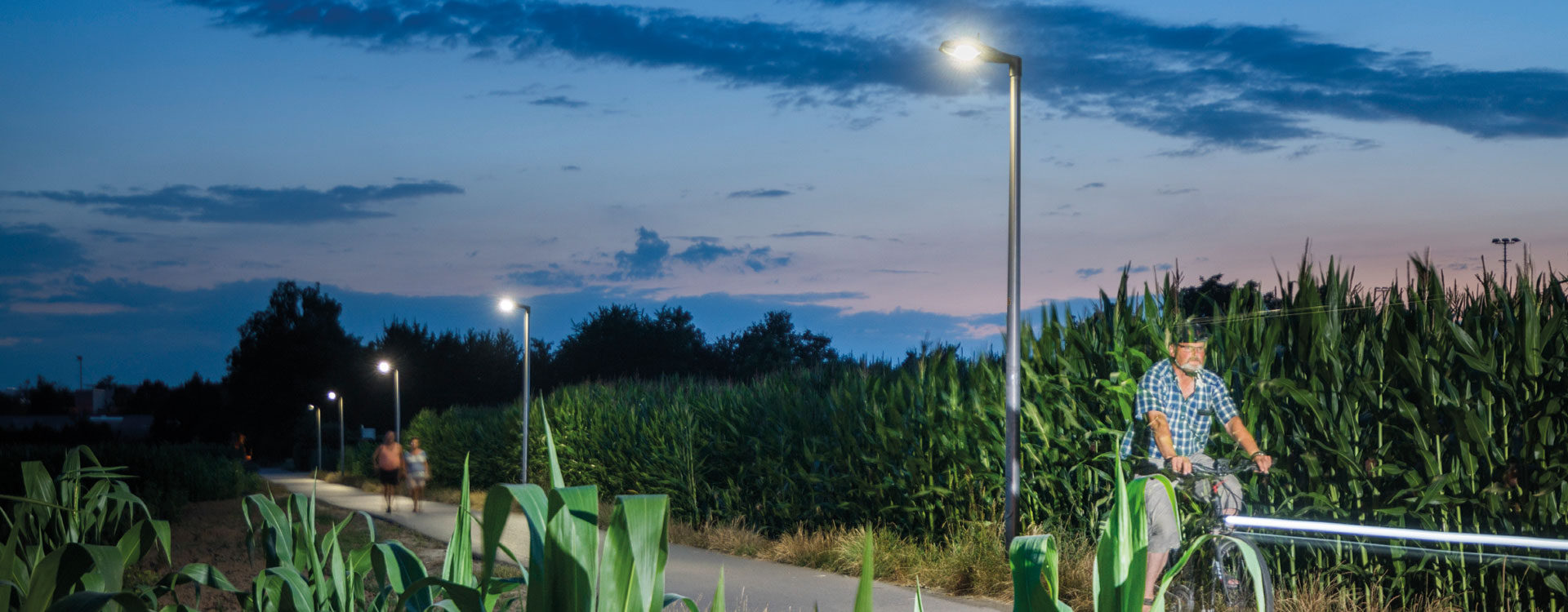This live-action photograph captures a serene evening scene along a lighted, paved path, just as the sun is setting. The sky is blue with clouds and gradually darkening, casting a dusky ambiance over the area. The path, illuminated by several security light poles, winds through a cornfield, with tall stalks of corn lining both sides. In the foreground, an older gentleman with a beard and goatee rides his bicycle, dressed in a striped shirt, shorts, and wearing a helmet. Behind him, two individuals walk at a distance; one in an orange sleeveless shirt and shorts, the other in a t-shirt and shorts. The scene depicts the quiet charm of a local path, used by walkers and cyclists alike, near a small town or city, emphasizing the peaceful transition from day to night. In the background, buildings are faintly visible, completing this tranquil snapshot of daily life.